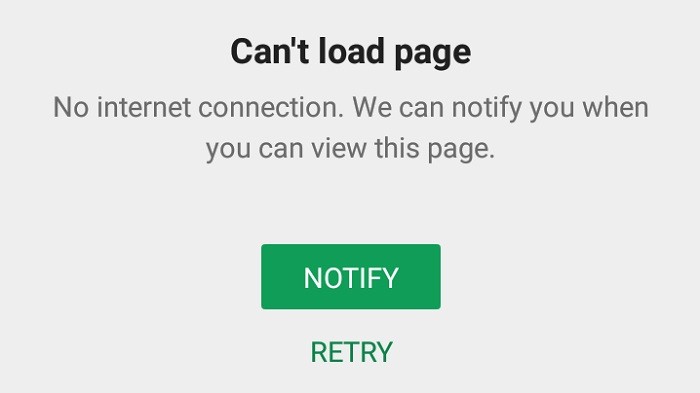The image depicts an error page on a gray background, indicating various potential issues such as a failed page load, server unavailability, or connection problems. The page is presented within a rectangular box. At the top center, bold black text states "Can't load page." Beneath this, lighter black or dark gray text reads, "No internet connection. We can notify you when you view this page." Further down, the page features two buttons. The top button is an emerald green color with rounded corners and the word "Notify" in white. Below it, the second button is a plain green box labeled "Retry."